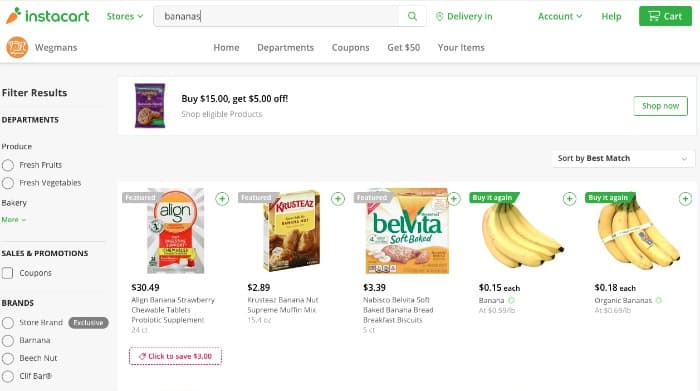This image showcases an Instacart interface. The upper left corner prominently features the iconic orange carrot logo and the word "Instacart" written in green. The interface is primarily set against a white background. 

At the top, there is a green drop-down menu for selecting different stores, and within the search bar, the word "bananas" is entered. Adjacent to the search bar, the text "Delivery in" is displayed in green, accompanied by a small location icon. To the right are options for accessing your account, a help section, and a green square button labeled "Cart" in white.

Results are neatly filtered by departments, including options for 'Produce,' 'Fresh Fruits,' 'Fresh Vegetables,' 'Bakery,' and more. There is also a section for 'Sales and Promotions' and another for 'Coupons,' which features a small checkbox. The brands available for selection include 'Store Brand,' 'Banana,' 'Beech-Nut,' and 'Clif Bars,' with store brands marked by a yellow label that seems to indicate "Exclusive."

The center of the image highlights a promotional message: "Buy $15, get $5 off" when shopping eligible products. Below this, various product options like 'Align,' 'Krysta's,' 'Belvita,' and items typically categorized as breads or chips are displayed. Notably, there are two distinct sections for bananas, each offering a ‘Buy Again’ option encapsulated in a green square at the top.

All listed items are accompanied by a small plus symbol for easy addition to the shopping cart, and at the bottom, there’s a coupon section inviting you to "Click to save $3."